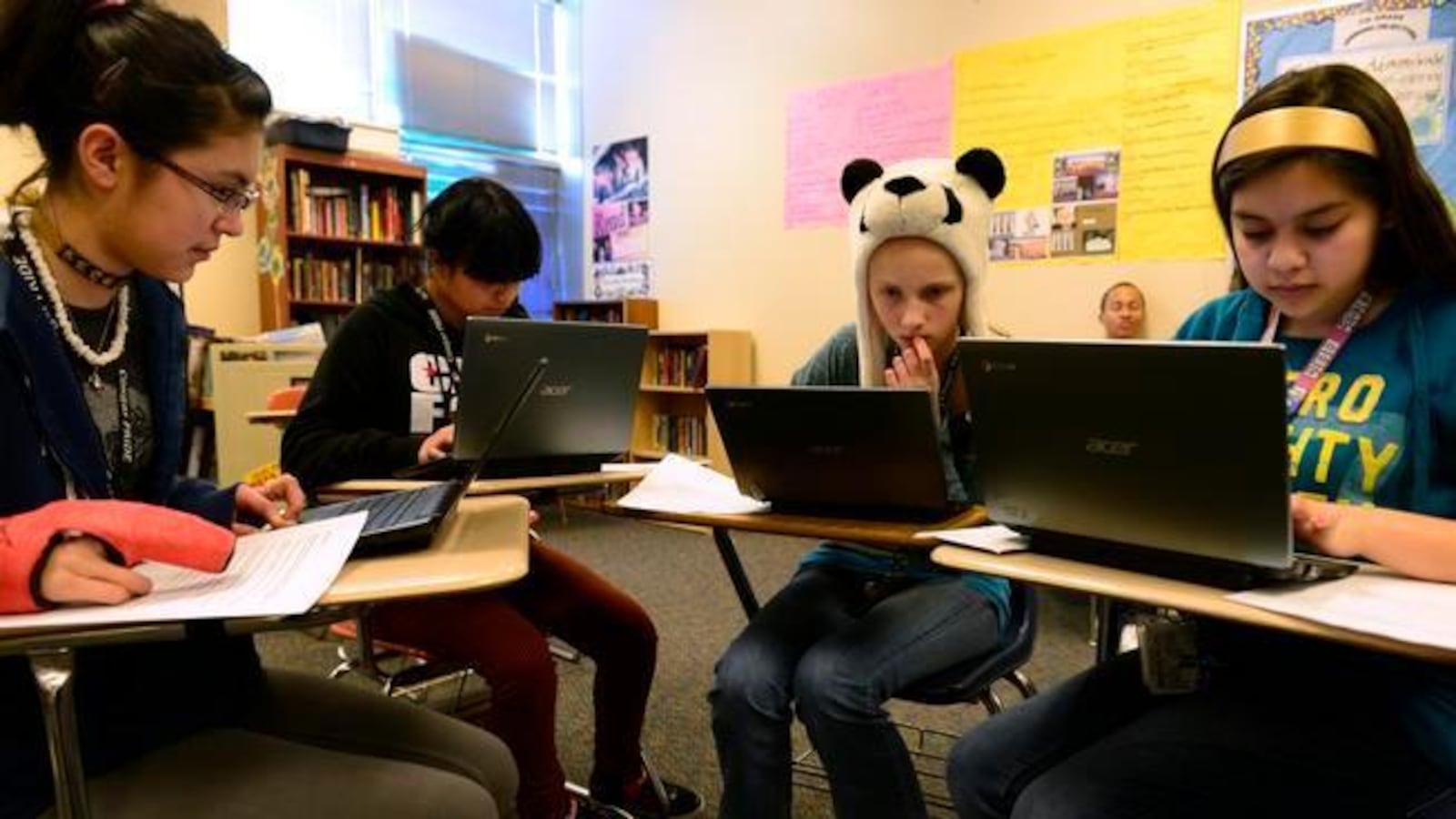In this image, a group of middle school students are in a typical classroom setting. The focal point is four students arranged in a V shape, engrossed in their studies while seated on half desks. From the left, there is a girl with glasses wearing a dark top and taupe pants, who also has a red cast on her right hand, suggesting a broken finger. She is using an Acer laptop, similar to the other students. Next to her is a boy with short hair, wearing a shirt and red pants, focused on his laptop. Beside him is a girl wearing a panda beanie, which adds a playful touch to her appearance. She is also dressed in jeans and using a laptop. On the far right, a girl with long hair adorned with a yellow headband can be seen. She is wearing a shirt with unreadable text and jeans, and she too is working on a laptop. In the background, there is an older student who seems to be sleeping, leaning against the wall. The classroom is decorated with bookshelves on the left and colorful posters on the right, enhancing the scholastic atmosphere.